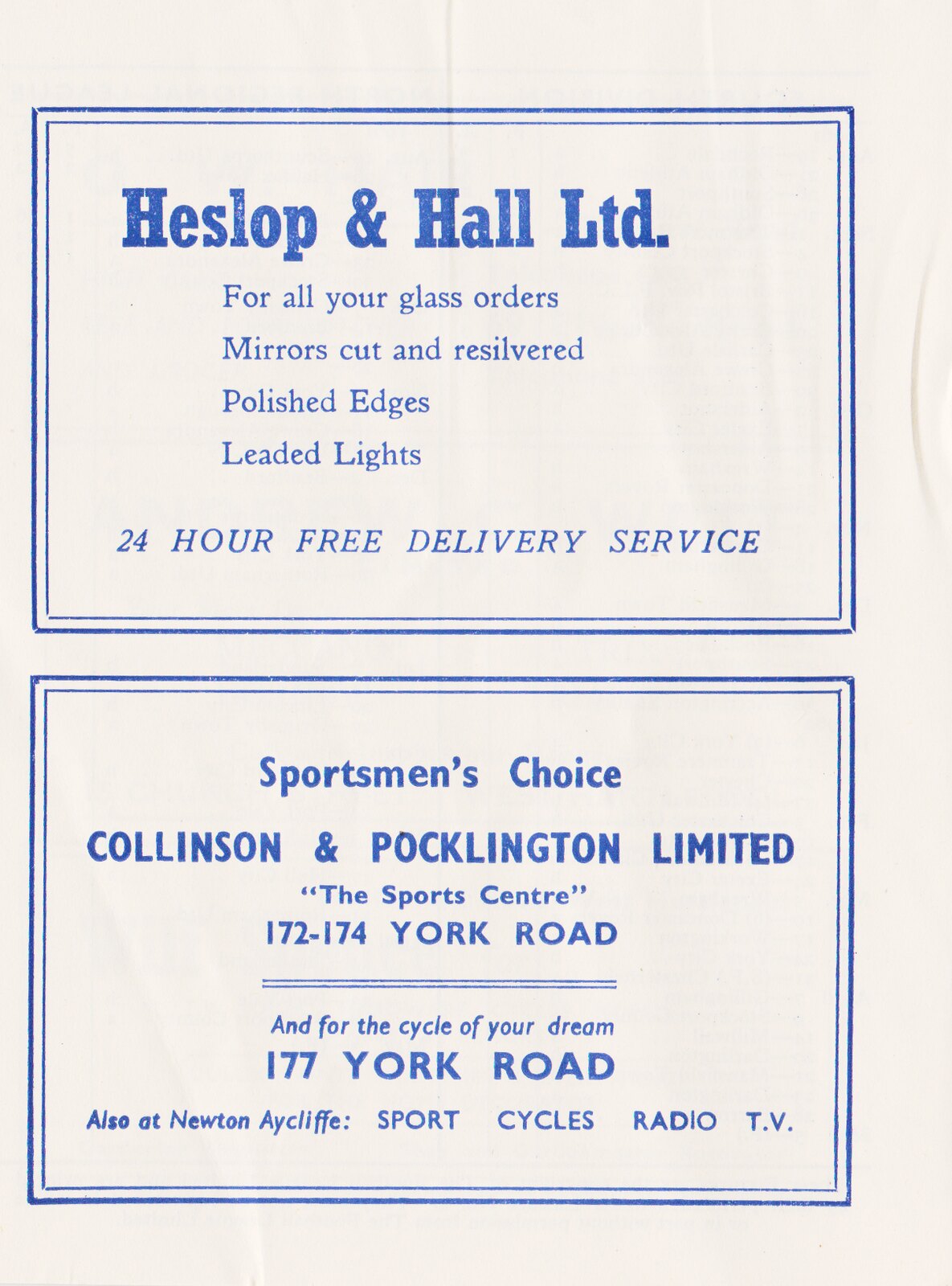The image depicts an old, slightly wrinkled, off-white piece of paper featuring blue text arranged in two rectangular advertisements. The top advertisement reads: "Heslop and Hall Limited - For all your glass orders: mirrors cut and re-silvered, polished edges, leaded lights, with a 24-hour free delivery service." This text is presented in a serif font. Below it, the second advertisement, in a sans-serif font, promotes "Sportsman's Choice, Collinson and Pocklington Limited," which includes information about "The Sports Centre" located at 172-174 York Road, "The Cycle of Your Dream" at 177 York Road, and "Newton Aycliffe Sport Cycles Radio TV." The careful arrangement and spelling, such as "Centre," suggest that these ads were likely part of a UK-based football club program or similar promotional material.